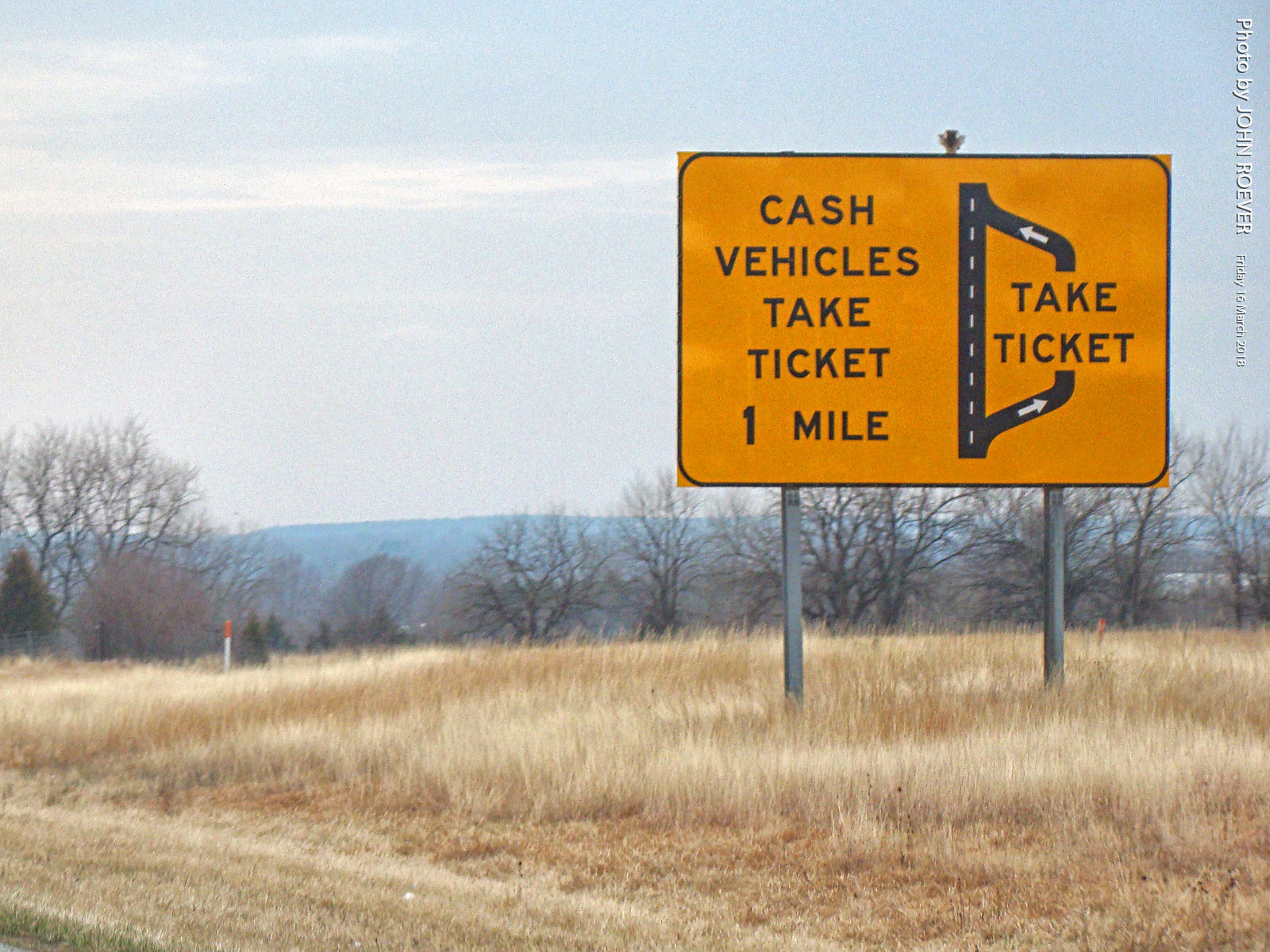This photograph features a large, orange road sign located on the side of a field with dead, tan-colored grass, indicative of late fall or winter. The deciduous trees in the background are barren, although some pine trees are visible. The sky is mostly cloudless but appears overcast, giving the scene a crisp yet muted quality. 

The sign, supported by two silver metal posts, has a yellow rectangular shape with rounded edges and a thin black border. It displays black text that reads: "Cash vehicles take ticket one mile." On the right side of the sign, a diagram illustrates a road diverging to the right with arrows directing vehicles to "take ticket," before converging back to the main road.

The image appears to be taken from within a vehicle and includes a photo credit along the right side that reads "Photo by John Rover," along with a date: Friday, March 15th or 16th, 2018. The distant background of the photograph features subtle mountainous terrain, enhancing the depth and setting of this toll road advisory scene.